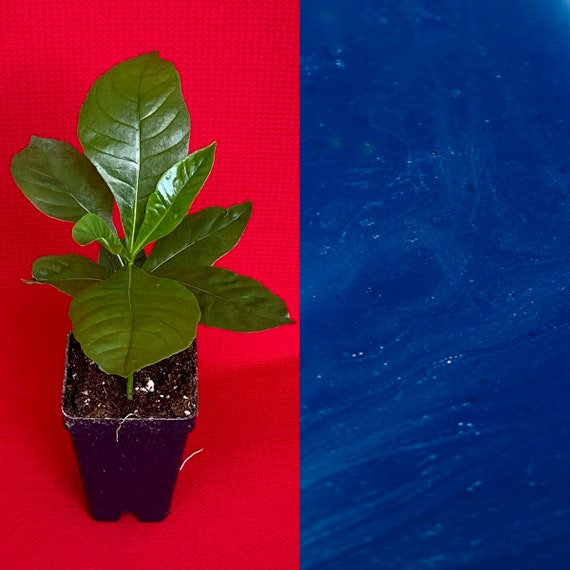The image is divided into two distinct halves. On the left, a young, recently potted plant sits in a plain black plastic container filled with soil. The background is a vibrant, almost duct tape-like red. The plant, with several shiny, deep green leaves featuring prominent veins, rests on an unspecified surface. On the right, the image displays a rich, deep blue side that resembles marble, with various shades of royal blue interspersed with white striations, giving it a watery, swirling look. The contrast between the left's vivid red and green against the right’s elegant blue marble creates a striking visual juxtaposition.